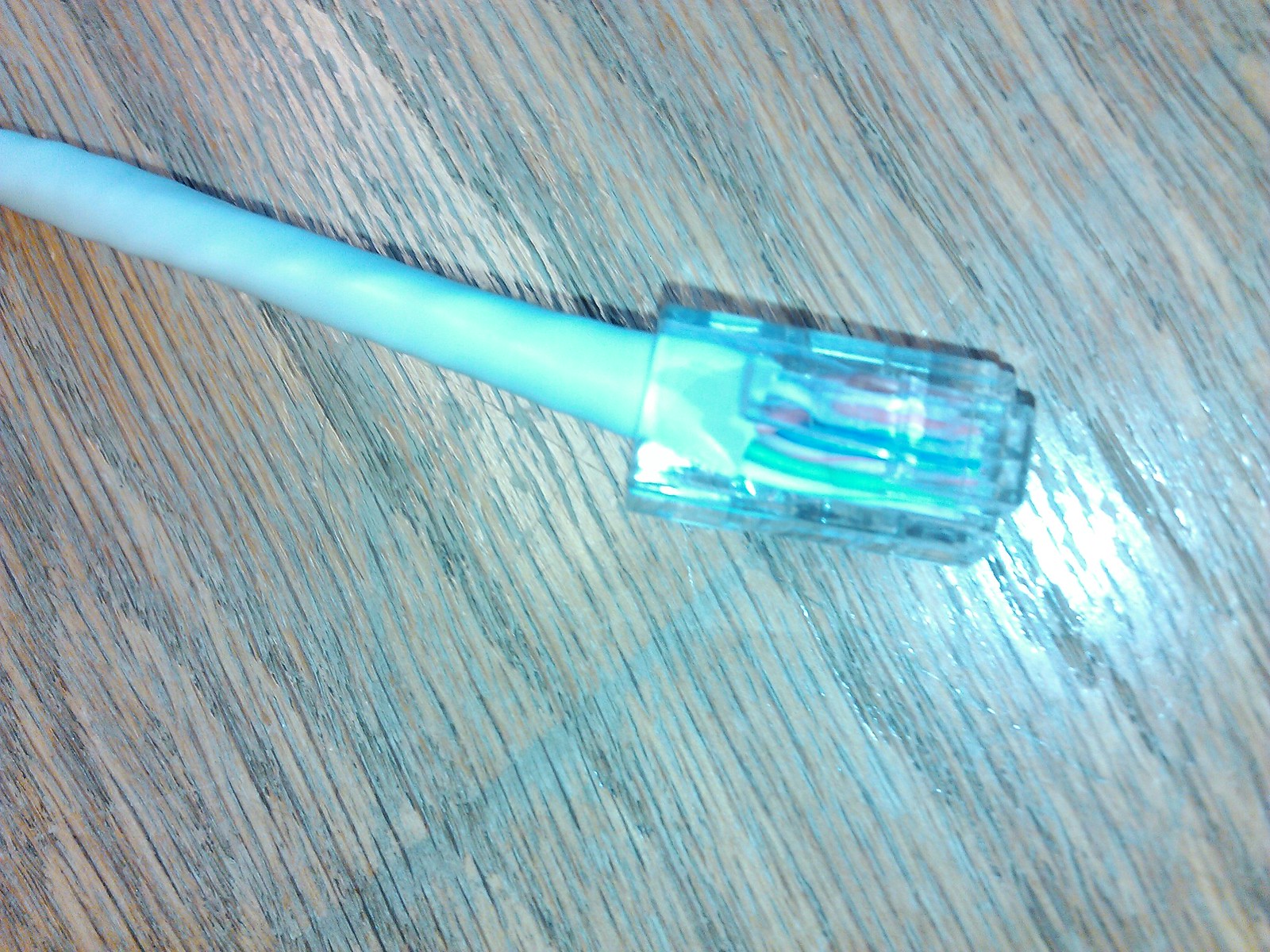The image is a close-up photo of an Ethernet cable on a wooden table. The Ethernet cable has a clear, translucent plastic connector at its end, through which various tiny wires—green, blue, white, and red—are visible. The cable itself appears to be off-white or light green, and it extends from the top right-hand side of the image towards the center. The wooden table has a dark, grooved texture, and there is a light source illuminating the right side of the image.